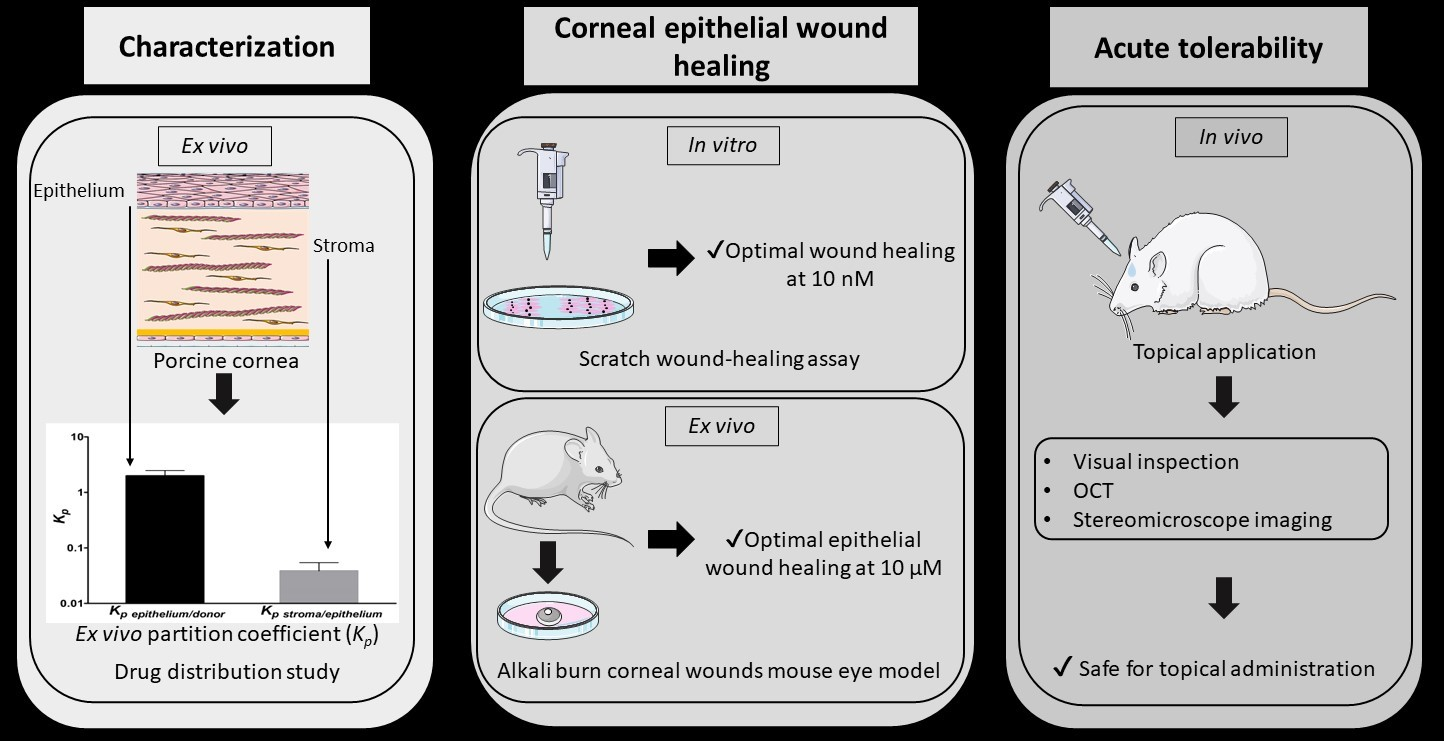The image is a detailed scientific diagram on a black background, divided into three sections, each with a gray box and labeled at the top. The first section, "Characterization," features images labeled "epithelium and stroma," "porcine cornea," and terms such as "ex vivo partition coefficient," "Kp," followed by a bar chart labeled "drug distribution study." The middle section, "Corneal Epithelial Wound Healing," is split into "in vitro" and "ex vivo" subsections, showing an image with something dripping into a Petri dish and mentioning "optimal wound healing at 10 nm," "scratch wound healing assay," "optimal epithelial wound healing at 10 µm," and "alkali burn corneal wounds mouse eye model," with an image of a mouse. The third section, "Acute Tolerability," includes images of a dropper applying something to a mouse, labeled "topical application," followed by "visual inspection," "OCT," "stereo microscope imaging," and "safe for topical administration." The diagram visually conveys the process and results of drug testing on mice, emphasizing wound healing and safety assessments for topical applications.